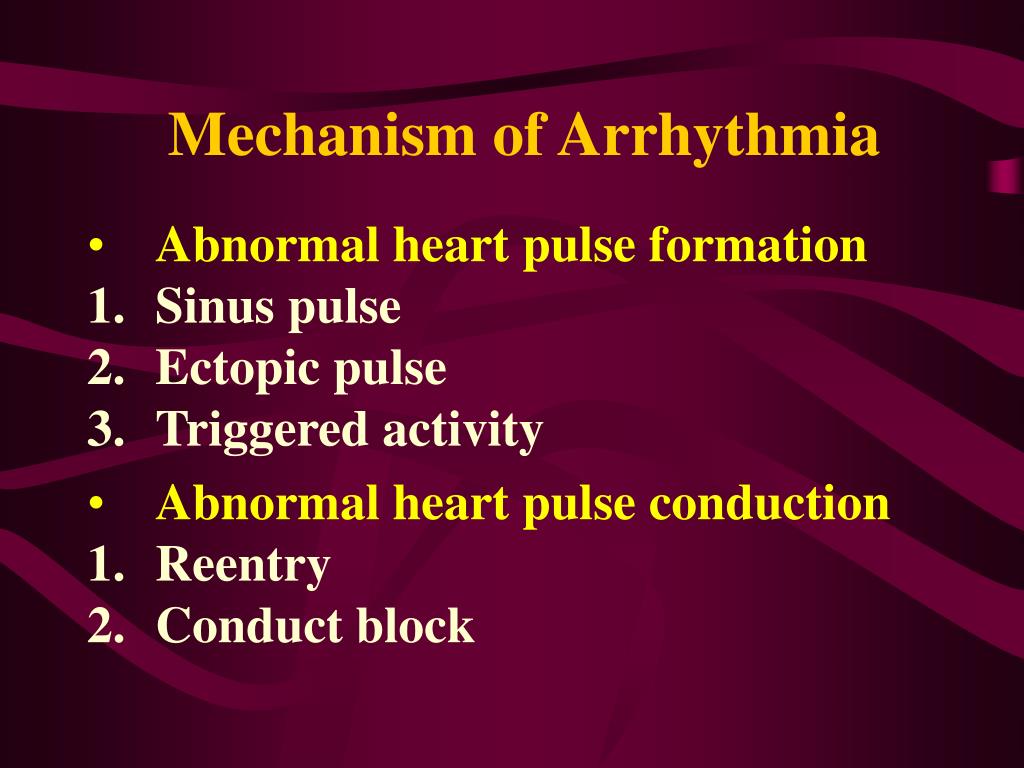The image resembles a Google Slides or PowerPoint presentation slide focused on the "Mechanisms of Arrhythmia." The background features various shades of purple, ranging from dark to light, interspersed with wavy lines. At the top, there is a yellow-orange title text, slightly larger than the rest, that reads "Mechanisms of Arrhythmia." Below this, the content is organized with bullet points and numbered items. The first bullet point in yellow text states "Abnormal Heart Pulse Formation," followed by three numbered items in white text: 1. Sinus Pulse, 2. Ectopic Pulse, and 3. Triggered Activity. Another yellow bullet point below this reads "Abnormal Heart Pulse Conduction," followed by two numbered points in white text: 1. Re-entry and 2. Conduct Block. The entire layout is presented in a rectangular format from left to right.